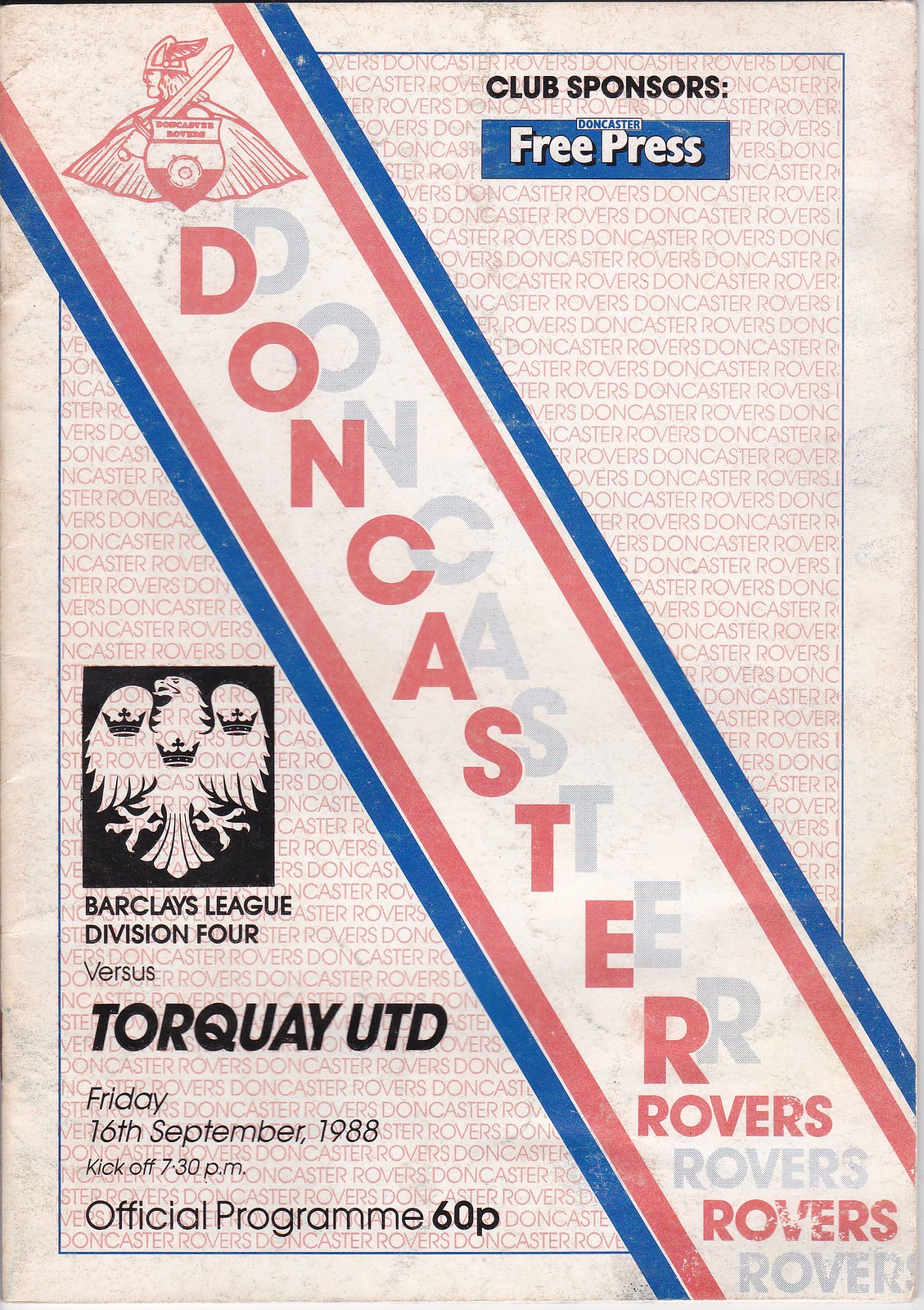The image is the front cover of an old, faded sports program or magazine for a Doncaster Rovers match. The cover is printed on an off-white piece of paper with a blue border framing the main content. The background inside this blue border features a red pattern formed by the words "Rovers Doncaster" repeated over and over. Diagonally from the top left to the bottom right run five bars: a thin blue bar, a thin red bar, a much thicker white bar, another thin red bar, and finally a thin blue bar. 

In the center of the cover, the words "Doncaster Rovers" appear in white text, overlaid on an orange border. At the top left corner is the Doncaster Rovers logo, featuring a Viking with a sword and shield. Just below it, the text reads "Club Sponsors, Doncaster Free Press." On the left side of the cover, "Barclays League Division 4" is noted with a logo above it. Beneath this, the text reads, "Versus Torquay UTD, Friday, 16th, September, 1988, kickoff, 7.30pm." In the bottom left corner, an image of an eagle with three crowns inside it sits above the text, "Official Program, 60P."